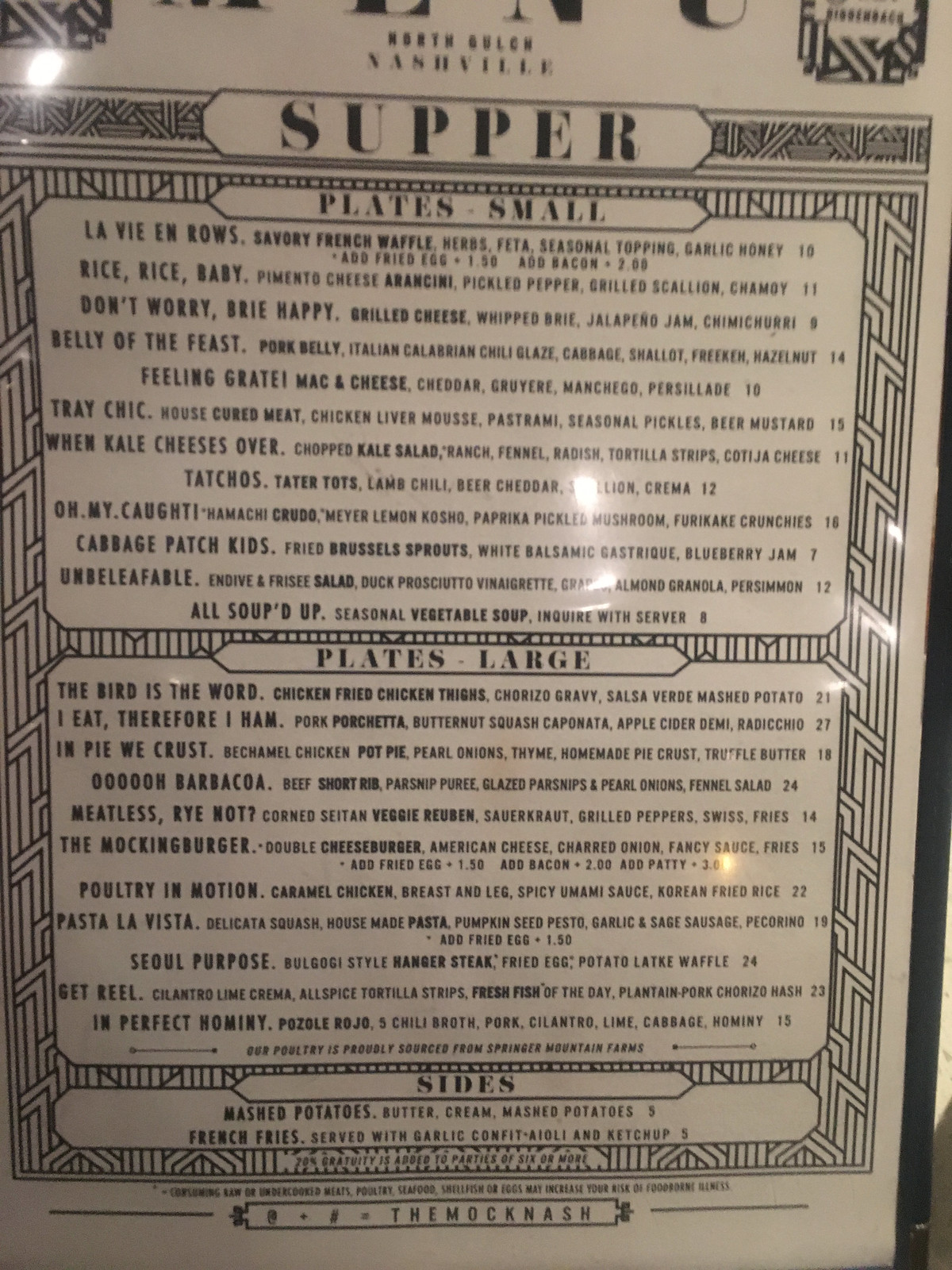The image depicts a slightly blurry food menu titled "North Something," suggesting a North-themed eatery located in Nashville. The menu features prominent headings such as "Supper" and is categorized into sections: "Plates Small," "Plates Large," and "Sides." The entire menu is presented in black and white and is partially framed in black, visible only on the right side. Each dish listed includes a description and price, such as "Don't Worry Pretty Happy," a grilled cheese sandwich with whipped brie, jalapeno jam, and chimichurri, priced at $9. At the bottom of the menu, there is a note indicating a 20% gratuity for parties of six or more, along with an allergen warning.